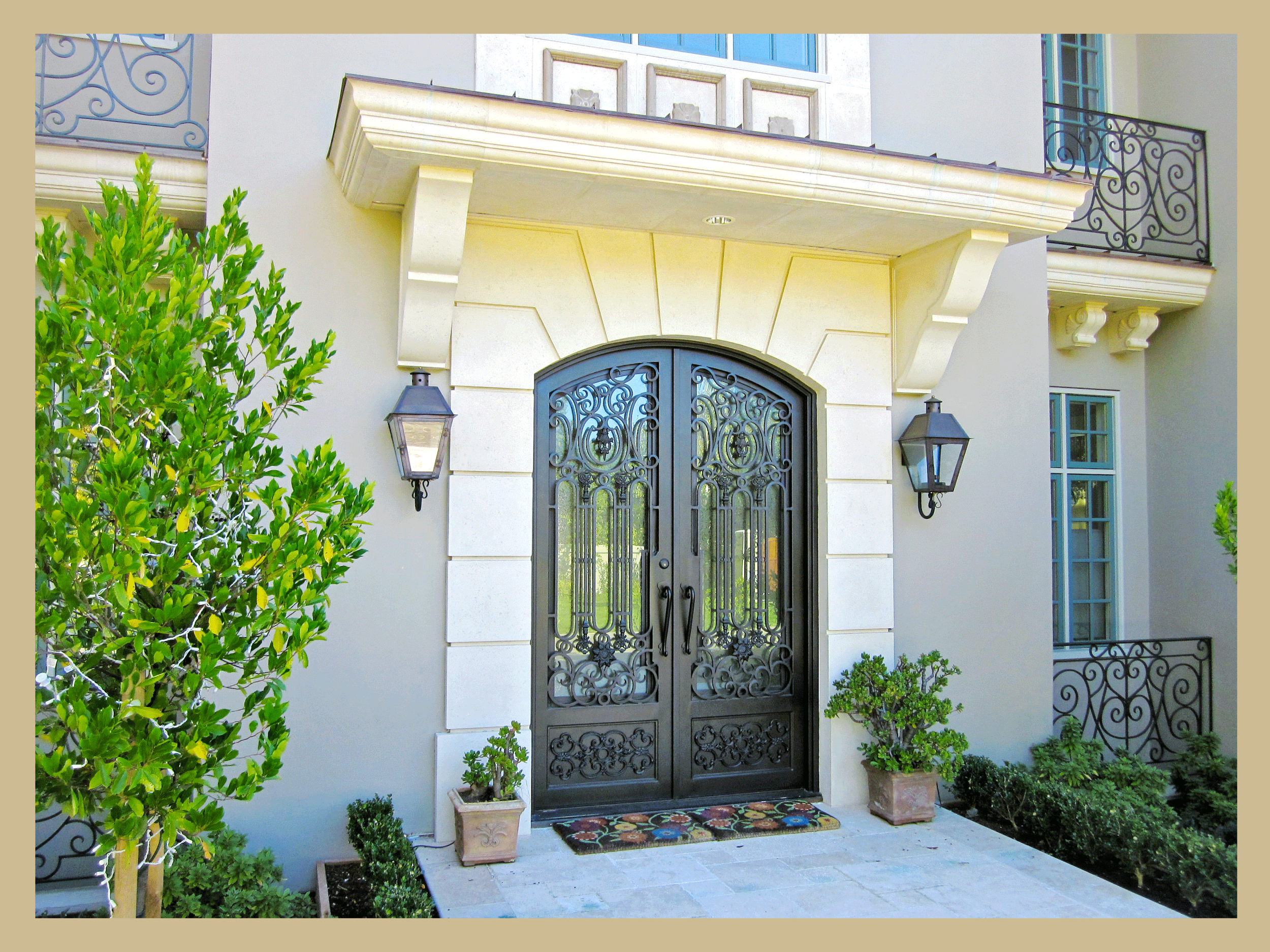This is a detailed photograph of the front porch of a two-story house. The central feature is a pair of large, dark brown double doors with wrought iron and glass detailing, each forming a slight arch at the top. These doors are surrounded by a pristine white facade, flanked by black metal lampposts. Above the doors is a decorative mantelpiece, adding to the regal and refined aesthetic of the entrance.

The walkway leading up to the porch is made of stone tiles, and welcomes guests with a black welcome mat adorned with multi-colored flowers. Directly in front of the doors are two potted plants, the one on the right noticeably larger, possibly a succulent or another type of leafy plant.

To the left of the pathway stands a mid-height green tree adorned with white Christmas lights, while on the right, just within the frame, is another tree. The bright and cheerful photo showcases additional greenery with small hedges at the bottom corners of the porch. The house itself is a sophisticated gray, and features several windows with wrought iron decorative covers, contributing to the overall elegant and inviting appearance of the home.